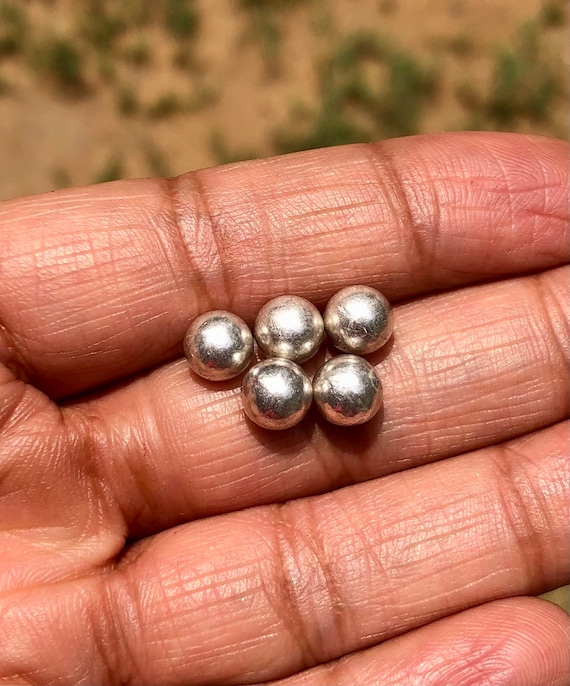The image is a detailed close-up of a tanned hand, specifically showing the index, middle, and ring fingers, with a faint glimpse of the pinky finger. The hand is facing upward with the fingertips pointing skywards. Notably, the person is holding five small, silver, worn balls with visible scratches, arranged with three on top and two on the bottom, positioned between the index and middle fingers. The background is a blurred mix of green and tan shades, suggesting an outdoor setting with dry ground and some greenery or shrubs.